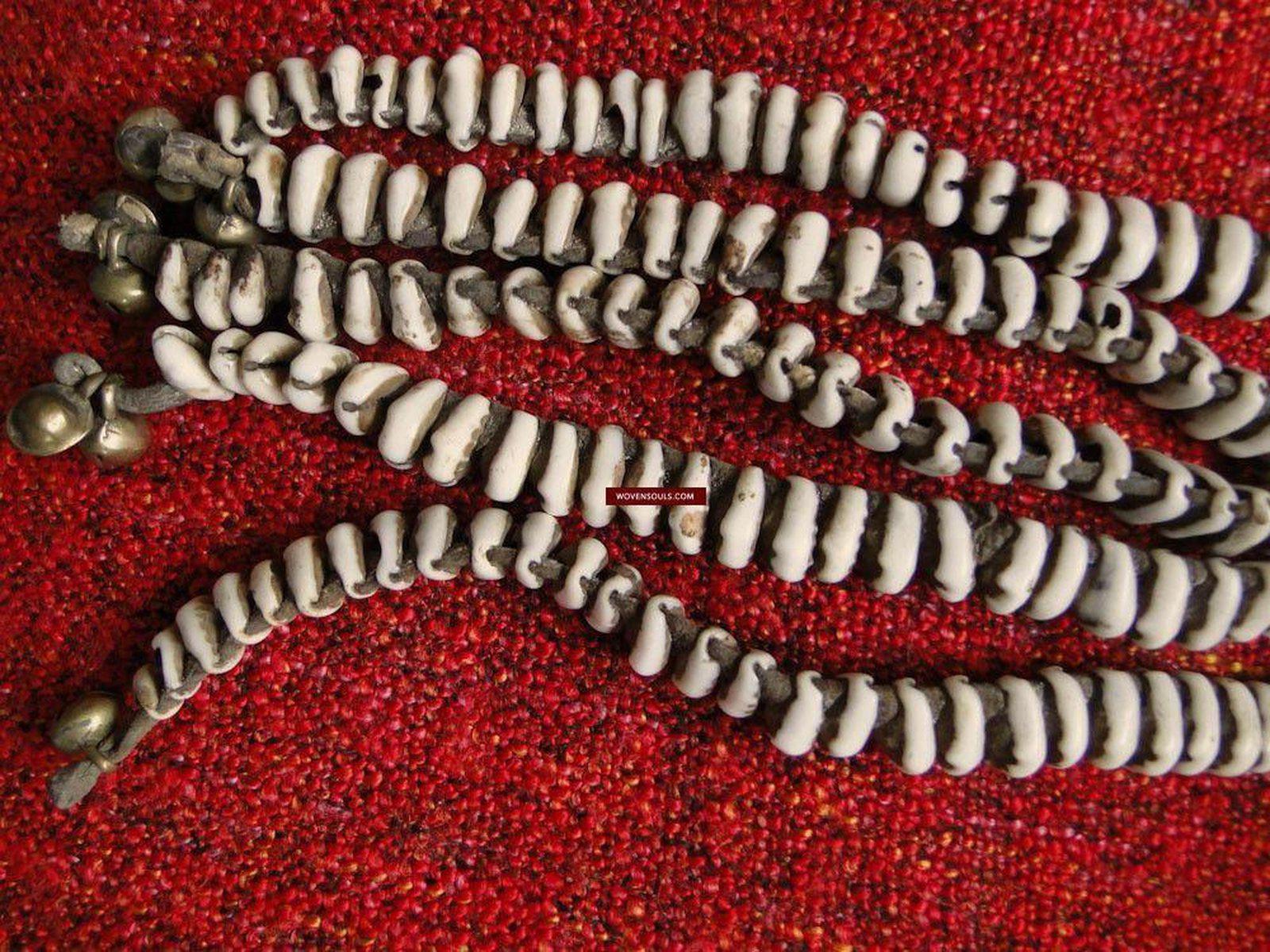The image depicts five pieces of what could be either bracelets or necklaces, arranged horizontally on a red woven fabric background. Each piece consists of a rope threaded with numerous circular, bead-like elements, varying in a creamy white to beige color. These elements may resemble small, polished stones or ivory-like beads, and each has a hole through the center for the rope to pass through. The ropes, brown in color, have one visible end on the left side, each adorned with a small, bell-shaped golden ornament. The arrangement is not perfectly straight; the strands exhibit slight and pronounced waves across their lengths. The right ends of the ropes are not visible in the image, making their full length undetermined.